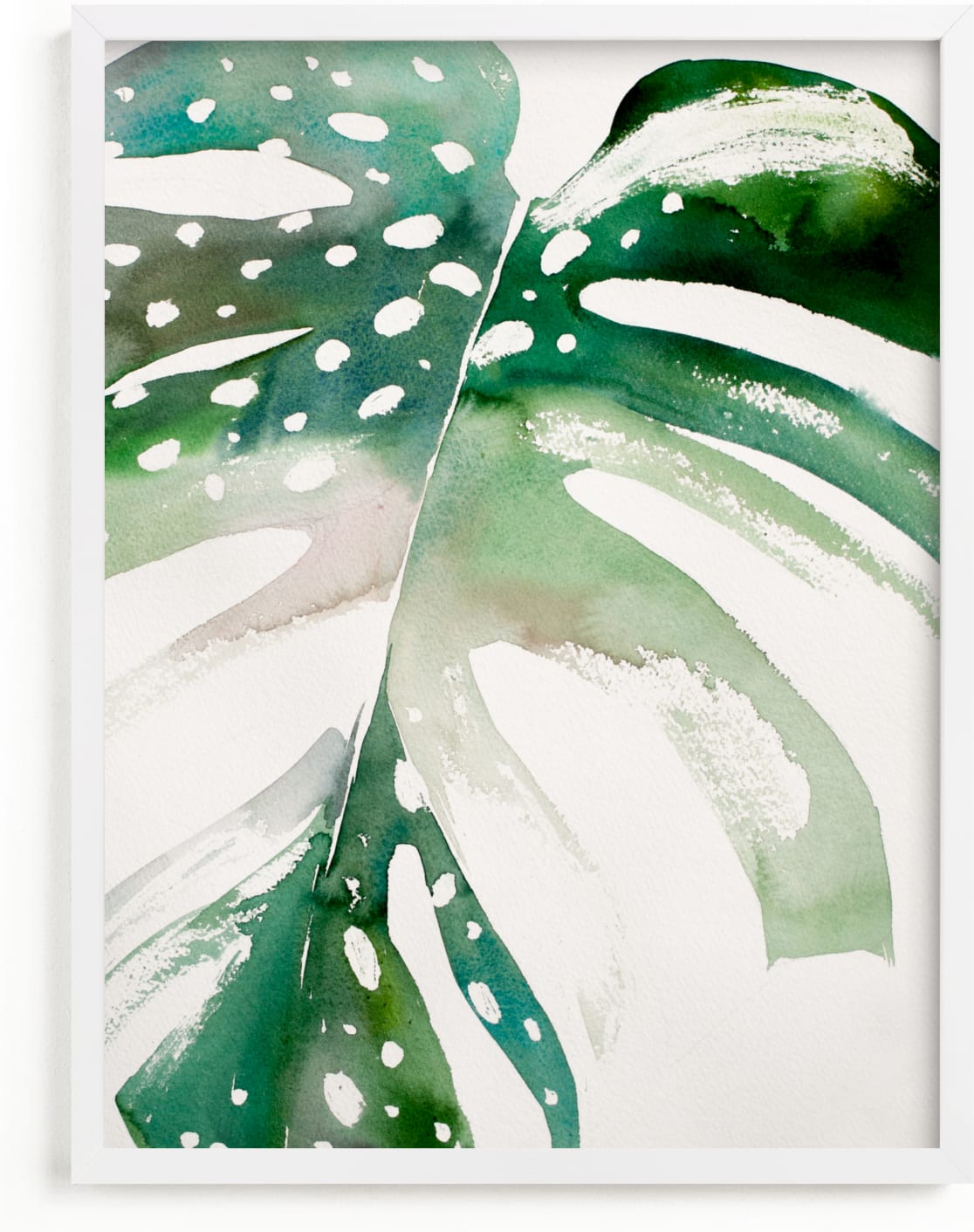The image is a framed abstract painting resembling a leaf, set against a white background. The central focus is a large, green leaf with a prominent vertical white line running through its middle, mimicking a leaf's central vein. The leaf features varying shades of green, from darker to lighter hues, and incorporates hints of pink on the left side of the central vein. Surrounding this main vein are green and white patterns, with some areas appearing to have been eaten by bugs or cut away, giving the painting a textured and layered feel. Numerous white dots are scattered across the leaf, predominantly on the larger leaves towards the top-left. Additionally, a brush of white highlights the brightest green leaf in the upper right, adding to the abstract nature of the art. The overall effect is enhanced by subtle shading, which creates a sense of depth and dimension.